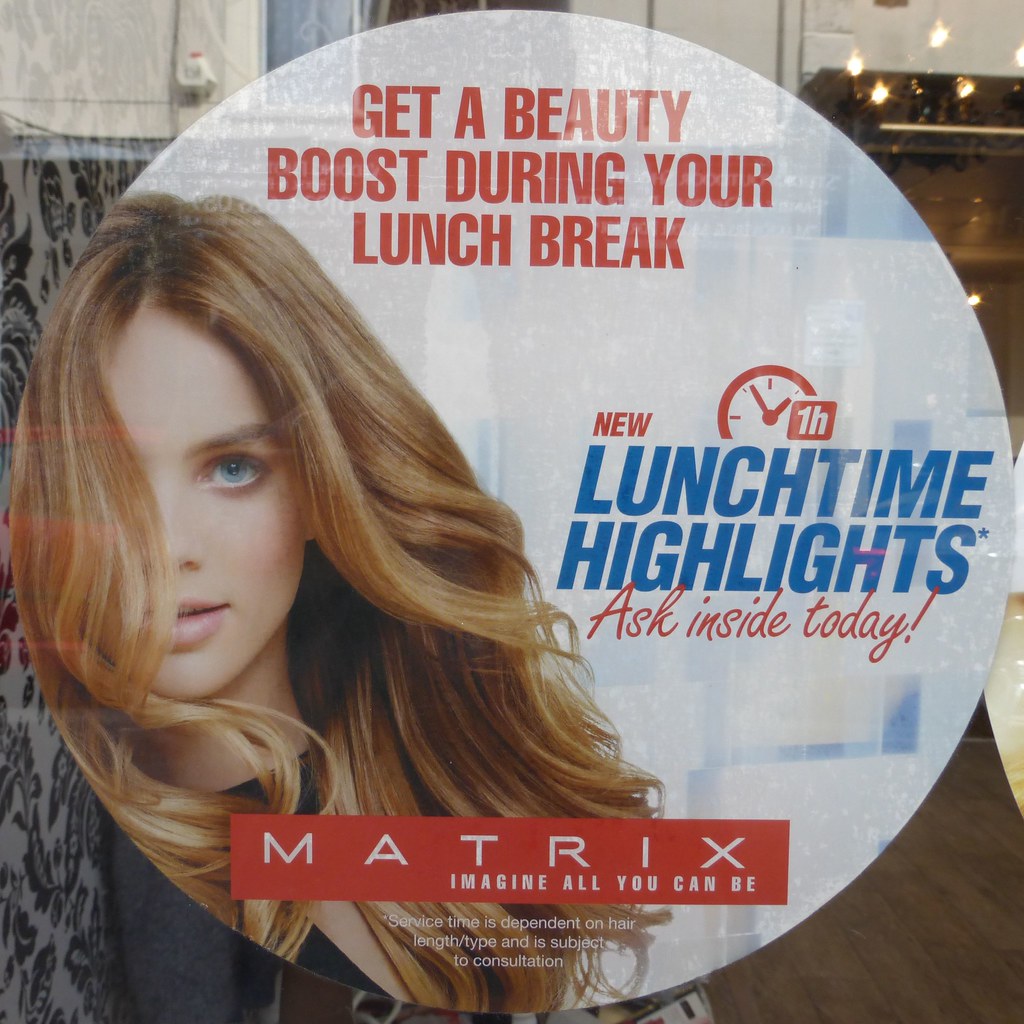The image features a circular advertisement prominently displayed behind glass, with reflections from the street visible. At its center is a striking model with flowing, wavy, blondish-brown hair, some of which cascades across her face. She has piercing blue eyes and a confident expression, gazing directly at the viewer with slightly parted lips. Dominating the top of the ad are bold, capital red letters that say, "GET A BEAUTY BOOST DURING YOUR LUNCH BREAK," accompanied by an icon of a clock indicating a one-hour duration. To the right of the model, it reads, "NEW LUNCHTIME HIGHLIGHTS." Below this, in elegant red script that isn't fully connected, the text invites, "ASK INSIDE TODAY!" At the bottom, the logo "MATRIX" appears in a sci-fi-like font with the tagline "IMAGINE ALL YOU CAN BE." A small disclaimer at the bottom notes that service time depends on hair length and type and is subject to consultation.